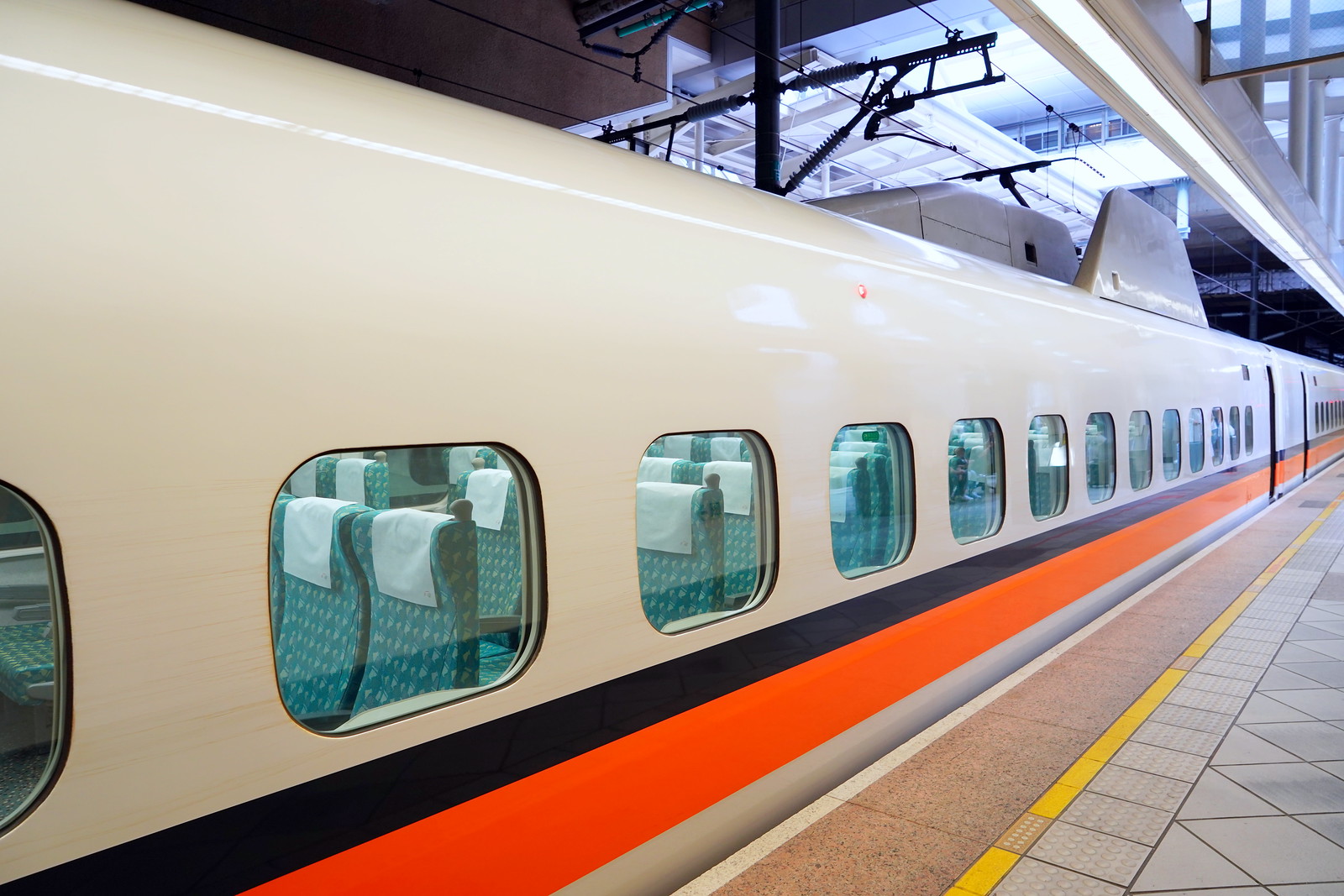This image depicts an electric subway train inside a station. The train extends from the top left of the frame, descending diagonally to the bottom left, then curving upwards to the middle right side of the image. The train's roof showcases the electrical wiring and mechanisms essential for its power. Below the roof, the train features numerous windows with a blue hue emitted from the cushioned blue seats arranged in multiple rows inside.

The exterior of the train is distinguished by its three-color scheme: a white top, a black stripe below the windows, and an orange stripe underneath that. The surrounding station structure includes visible beams and glass in the upper right part of the image, suggesting an indoor setting. The platform adjacent to the train is composed of red granite nearest to the train, followed by a thin yellow safety line, and finally transitioning to light gray tiles further away. There's also a light fixture situated above, illuminating the scene.